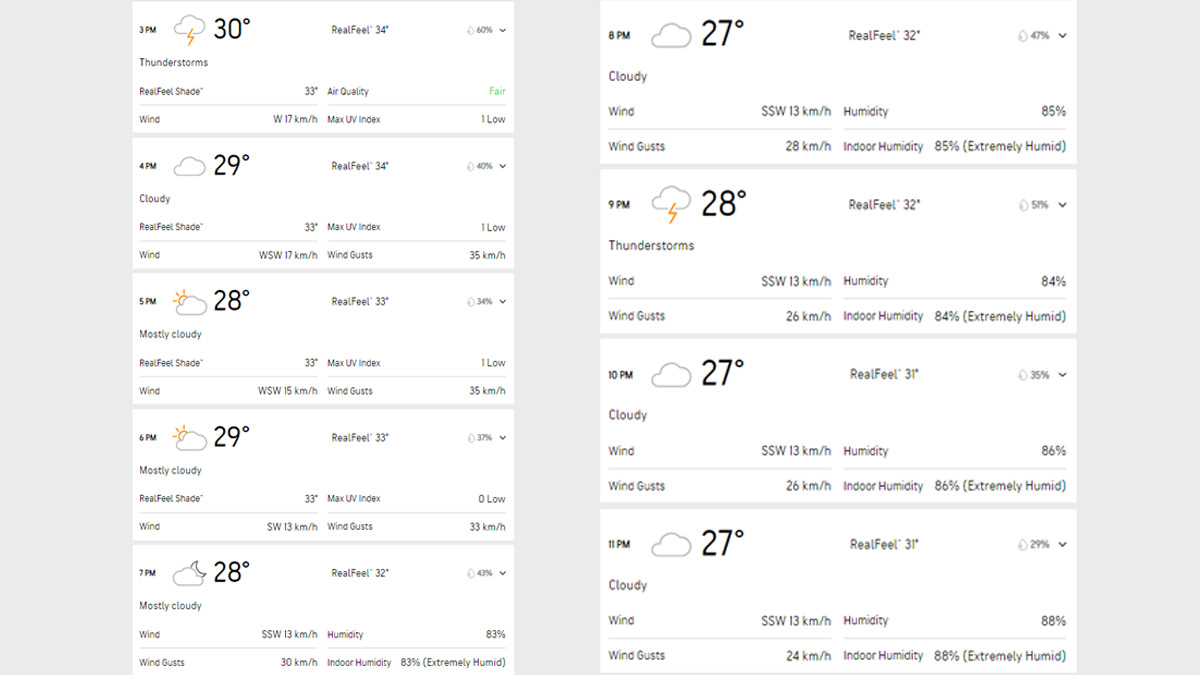In this image, we observe a detailed weather forecast divided into two vertical sections. The far-left section features a solid gray, vertically-oriented rectangle. Adjacent to it, on the right, there is a thicker white rectangular area, extending upwards. 

At the topmost part of this white section, it displays "30 degrees" with an icon of a cloud accompanied by a lightning bolt and the time indicated as "3pm." Just below that, the temperature reads "29 degrees" alongside a clear cloud symbol, labeled "4pm." Following this, the next segment shows "28 degrees" with a sun partly obscured by a cloud, marked as "5pm." Directly underneath, "29 degrees" appears again with a sun-and-cloud icon, tagged "6pm." At the bottom, it records "28 degrees" featuring a cloud and a moon, for "7pm."

The right section of the image continues with similar details. Starting from the top, it shows "27 degrees" with a cloud icon denoted for "8pm." The next tier lists "28 degrees" combined with a cloud and a thunderbolt symbol, likely indicating a storm, for "9pm." Below that, "27 degrees" with just a cloud is marked "10pm." Finally, the lowest segment records "27 degrees" again with a cloud for "11pm."

This composition clearly delineates the hourly weather conditions with respective temperatures and symbolic representations of the forecast, meticulously organized into two columns.